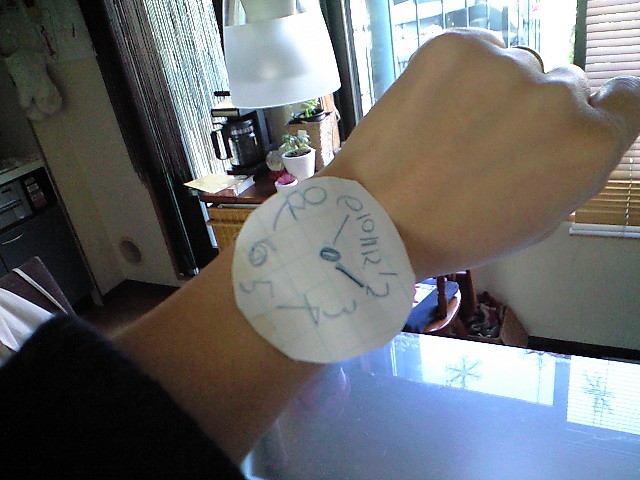In this color photograph, a person, possibly a man with a muscular forearm and a dark, possibly black or very dark blue, puffy sleeve that extends to the forearm, is prominently holding up their left wrist. The person's hand is clenched into a fist, showcasing the back of the hand and wrist. Taped to the wrist is a makeshift analog watch, evidently crafted by a child. It consists of a circle cut out from white graph paper, with imperfectly drawn numbers arranged haphazardly around the edge and positioned too closely together. The watch face includes a dot and two short lines representing the minute and hour hands. 

The background features a domestic setting with framed long windows, light filtering in through them. To the left of the image is a small brown table holding a coffee maker, while a large lamp with a white lampshade and three small potted plants can be seen behind it. On the right edge of the table is a piece of paper. A closer table, located in the foreground in front of the person, reflects light from the windows, adding a sense of depth to the scene. Additional household details include a pair of oven mitts hung on the upper left wall and a child’s drawing displayed on a thin wall to the right. The image encapsulates the contrast between the childlike simplicity of the handcrafted watch and the cozy, lived-in complexity of the surrounding room.